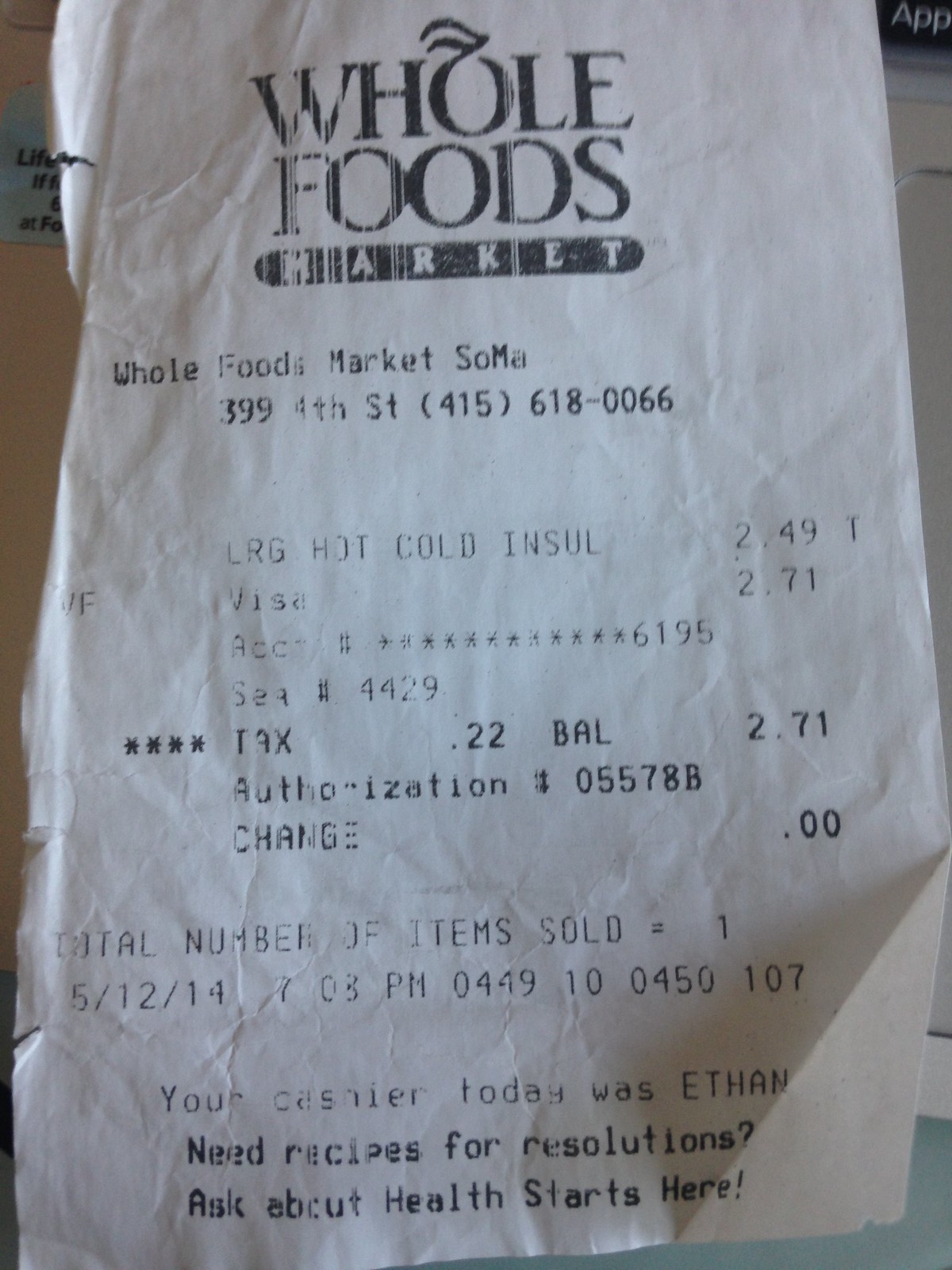This detailed and descriptive caption provides a comprehensive description of a store receipt from Whole Foods Market:

"Photograph of a Whole Foods Market store receipt. The receipt, printed on white paper, displays the 'Whole Foods Market' logo at the top in black. The 'O' in 'Whole Foods' features a leaf design, emulating an onion or tomato, and 'Market' is enclosed in an oval-shaped border with rounded ends. Below the logo, the store's address is listed as Whole Foods Market, Soma, 399 4th Street, with a contact number (415) 618-0066.

Itemized details follow, starting with 'L-R-G, hot, cold, IN-SUL, $2.49-T' indicating a purchased item. Payment information reads 'VF, Visa, $2.71', and account details are partially obscured, showing 'ACCT ######6195' and 'SEQ ####4429'. A note on tax lists '$0.22', and the final balance as '$2.71'. The authorization code is #05578B, and no change was given ($0.00).

The receipt concludes with the total number of items sold, notated as '1512-14703PM-0449100450107'. The cashier is identified as 'ETHAN' in all caps. Promotional information at the bottom suggests, 'Need recipes for resolutions? Ask about health starts here.'"